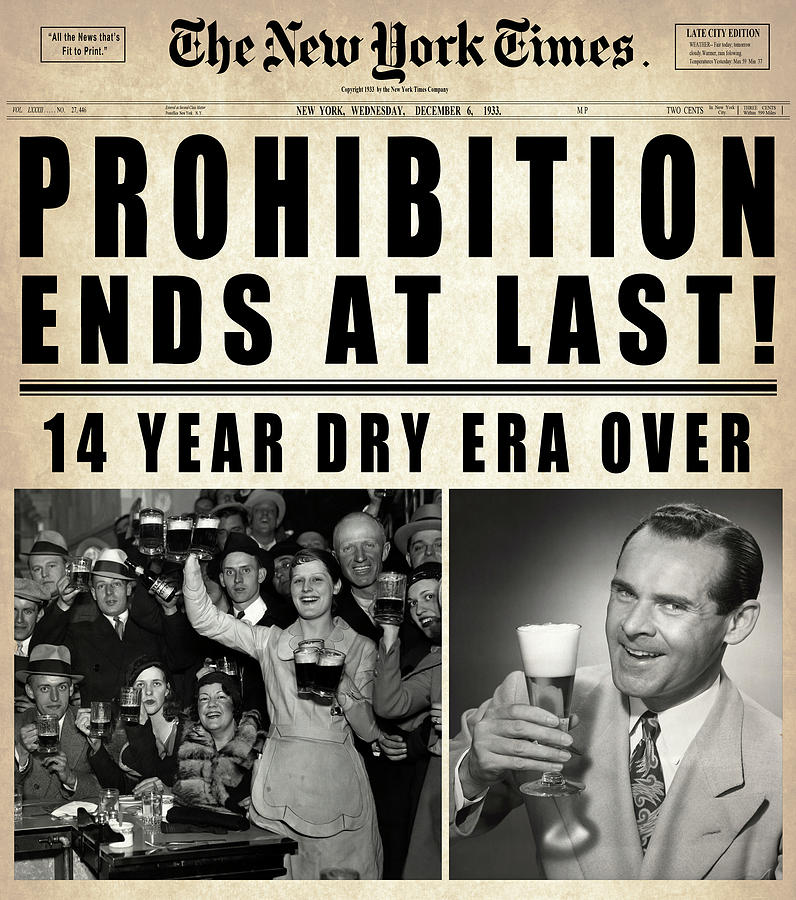This is a detailed photograph of the front page of the New York Times, dated Wednesday, December 6, 1933, priced at two cents. The aged and slightly tainted newspaper bears bold black letters announcing, "Prohibition Ends at Last!" marking the conclusion of the 14-year dry era. Below the headline, the description reads "14-year dry era over."

At the bottom of the page, two photographs capture the public's jubilant reaction to the news. On the left, a large group of approximately 20 people is seen in a bar, raising an assortment of beer glasses and mugs, with foam-topped dark beer visible. Most men in the group are wearing hats, and all appear cheerful and celebratory. On the right, an individual man dressed in a light-colored suit and tie holds up a Pilsner-style glass of beer, also with foam on top, while smiling broadly. The combination of these elements vividly captures the elation surrounding the end of Prohibition.